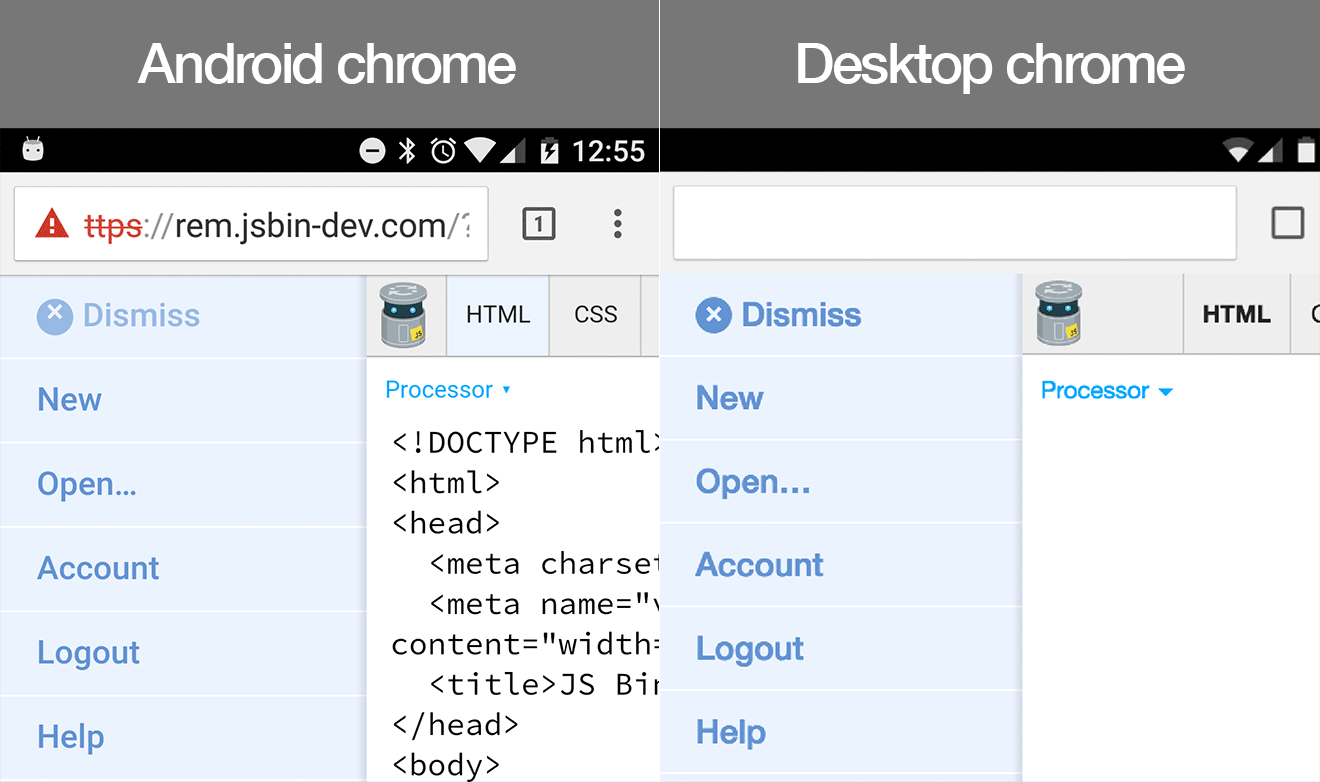The image is a detailed screenshot of an interface with specific elements highlighted. In the upper left corner, there is a gray header labeled "Android Chrome," while the upper right side displays the text "Desktop Chrome" in bold white letters. Directly beneath this, set against a narrow black background, are several icons: a whimsical face with antennae, a minus sign inside a circle, an alarm clock, a Wi-Fi symbol, a mobile reception indicator, a battery icon, and a time display reading 12:55.

The address bar in the screenshot reads "https://rem.jsbindev.com". On the left side, there is a navigation bar with the following labeled options listed vertically: Dismiss, New, Open, Account, Logout, Help. This same set of options is mirrored on the right side of the interface, appearing inside a light blue box with dark blue text: Dismiss, New, Open, Account, Logout, Help.